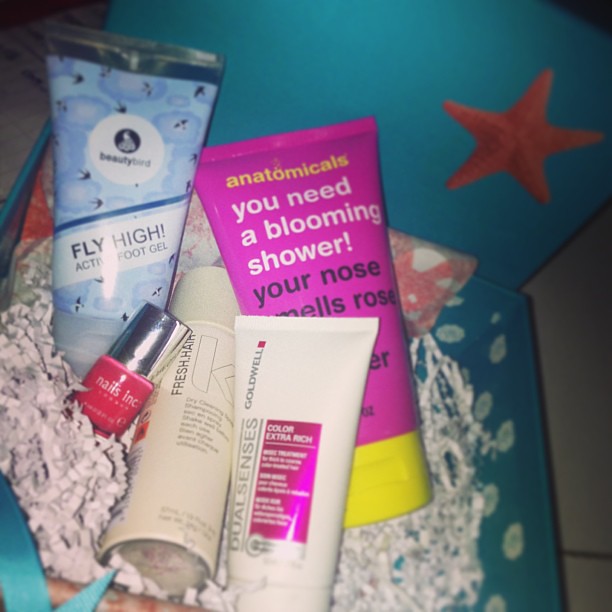The image depicts a collection of health and beauty products arranged in a vibrant blue cosmetic box adorned with a starfish on the inside upper lid. The items include a beige spray bottle labeled "Fresh Hair Spray" with a distinguishable "K" on it, a red nail polish, and a hot pink squeeze bottle that intriguingly states, "Anatopicals: You Need a Bloomy Shower. Your Nose Smells Rose." Another squeeze bottle, labeled "Dual Senses Goldwell Color Extra Rich," is presumed to be hair coloring. At the top, there's a bottle of "Beauty Bird Fly High Active Foot Gel." The contents are supported by confetti, reminiscent of celebratory filler, ensuring they remain secure. The box is situated in a dimly lit room, adding to the cozy and intimate presentation of these assorted cosmetics.